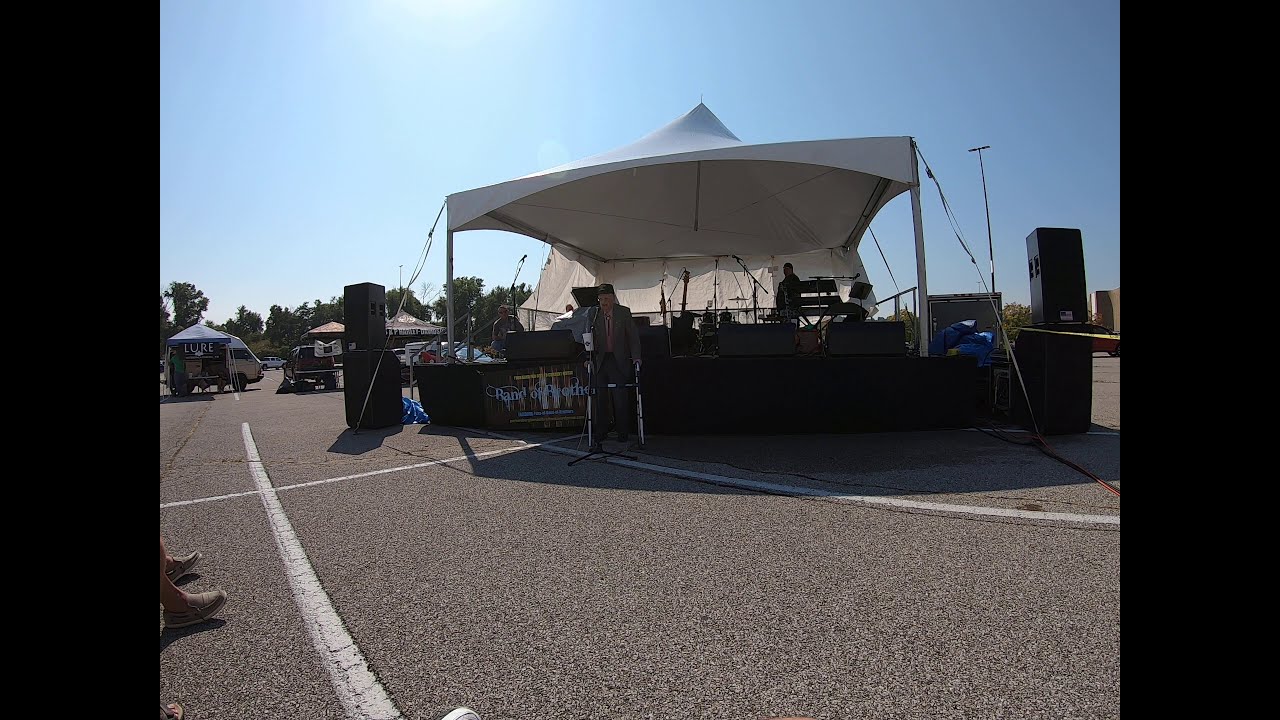The color photograph captures a lively outdoor event, likely a fair or craft show, set in a spacious, dark gray parking lot with white striping. Central to the image is a large white pavilion-type tent bearing a "Band of Brothers" sign. The tent houses a black stage equipped with various musical instruments and speakers stacked on either side. In front of the stage, an elderly man with a walker is seen speaking into a microphone, engaging the audience gathered at tables nearby.

Surrounding this main tent are several smaller tents, including one with a blue top and a sign that reads "Lure." These tents, along with some parked vehicles, are arranged against the backdrop of a clear blue sky devoid of clouds. The background also features leafy green trees, adding a touch of nature to the bustling scene. The overall atmosphere is bright and inviting, with the sunlight illuminating the entire area, capturing a vivid moment of community and entertainment. The photograph is presented in a landscape orientation, subtly framed by vertical black stripes on either side.